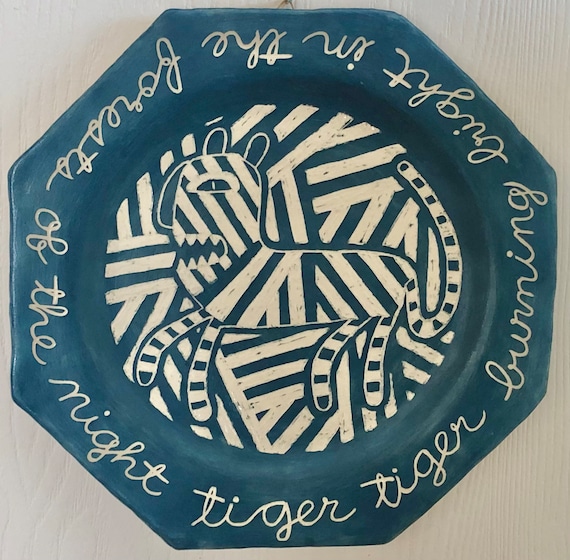This image depicts a dark blue, octagonal ceramic plate, resting on a light tan, wooden table with vertical grains. The plate, though predominantly octagonal, has slightly uneven edges giving it a handmade appearance. At the center of the plate is a vague yet striking depiction of a tiger, facing left with noticeable sharp teeth and diagonal stripes, both on its body and in the background. The simplistic, almost childlike design of the tiger is done in contrasting diagonal blue and white lines, contributing to a tribal-like aesthetic. Surrounding the tiger, in a circular pattern along the plate’s edge, is a cursive inscription in white that reads, "Tiger, tiger, burning bright, in the forest of the night." The artistic piece combines a primitive charm with an evocative depiction, marrying form and poetry seamlessly.